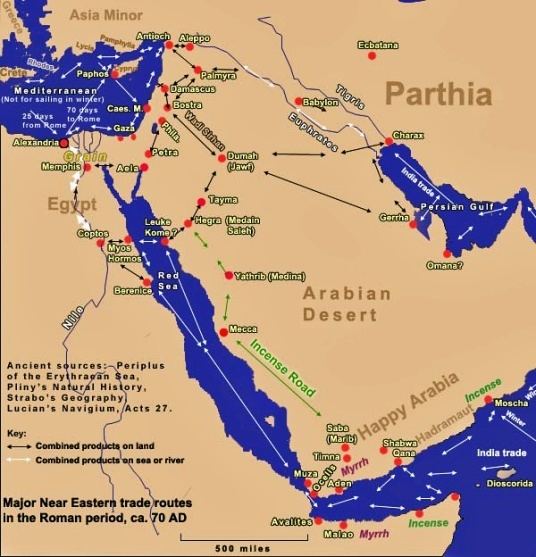This image is a detailed map of the Middle East during the Roman period around 70 AD, emphasizing major Near Eastern trade routes. Notable regions such as Parthia, the Arabian Desert, Egypt, and Asia Minor are prominently featured. The map includes a wealth of text highlighting major cities, including Memphis, Alexandria, Kaptos, Mecca, Hagra, Ghara, Omana, Babylon, and Ecbatana. In the lower part of the map, specifically in the region labeled "Happy Arabia," green arrows depict the Incense Road, illustrating the trade of incense, myrrh, and other goods along the Arabian Desert down to the bottom of the map. Key locations like the Red Sea, Mediterranean Sea, and the Persian Gulf are also identified. There's a key at the bottom left corner with black arrows indicating the trade routes of combined products on land and white arrows for routes on sea or river. Furthermore, a section in the bottom left corner lists ancient sources, including the Periplus of the Erythraean Sea, Pliny's Natural History, Strabo's Geography, Lucian's Navagum, and Acts 27. The map provides a comprehensive overview of trade dynamics in this historic period.